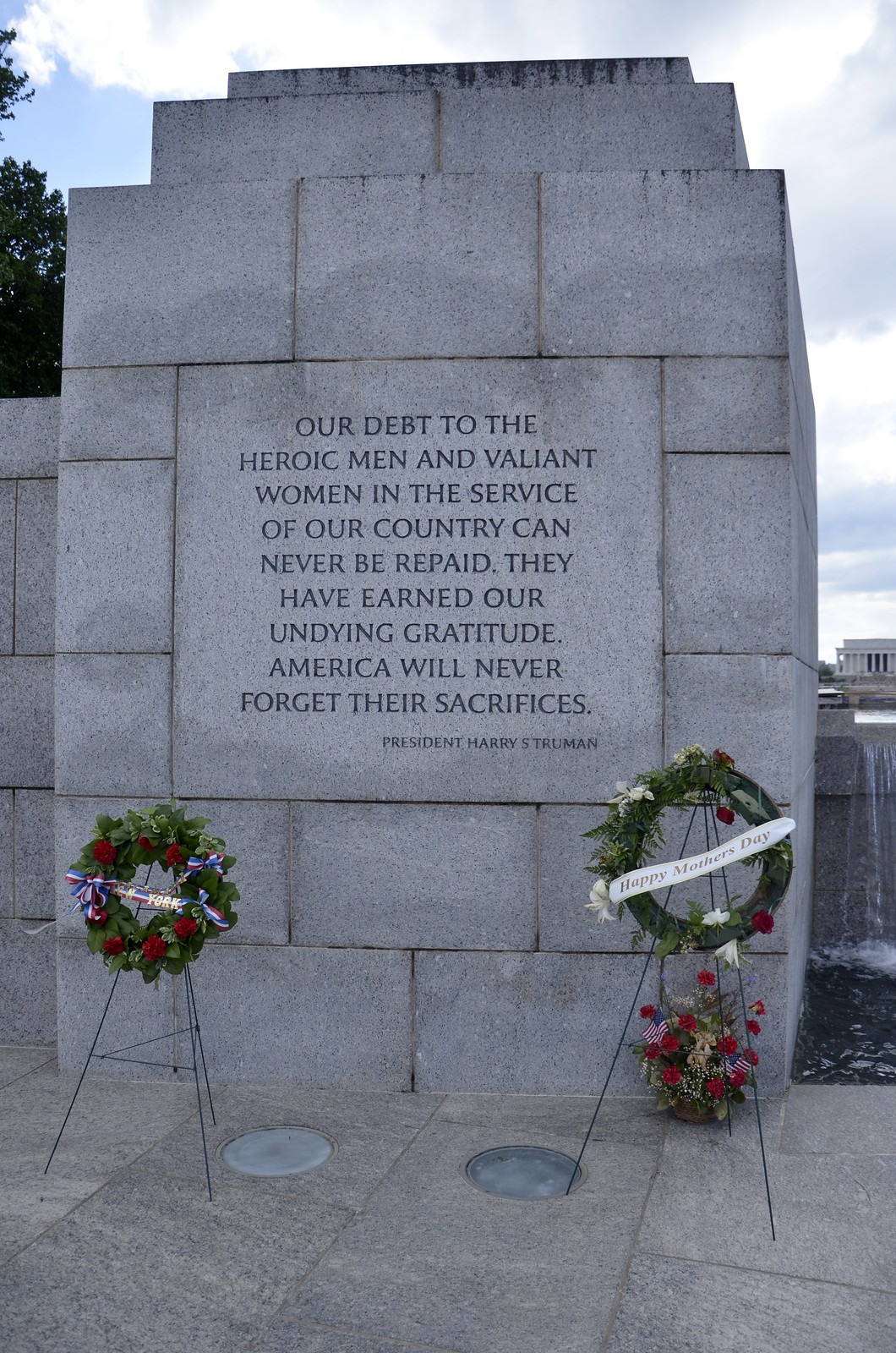The photograph features a memorial wall made of grey stones meticulously organized in rectangular and square patterns. At the center of the wall, a prominent square-shaped stone bears an inscription that reads, "Our debt to the heroic men and valiant women in the service of our country can never be repaid. They have earned our undying gratitude. America will never forget their sacrifices. President Harry S. Truman." In front of this solemn epitaph, there are two wreaths laid on the ground—one labeled "New York" and the other inscribed "Happy Mother's Day." The scene is set under a blue sky filled with clouds, adding a serene backdrop to this poignant tribute.